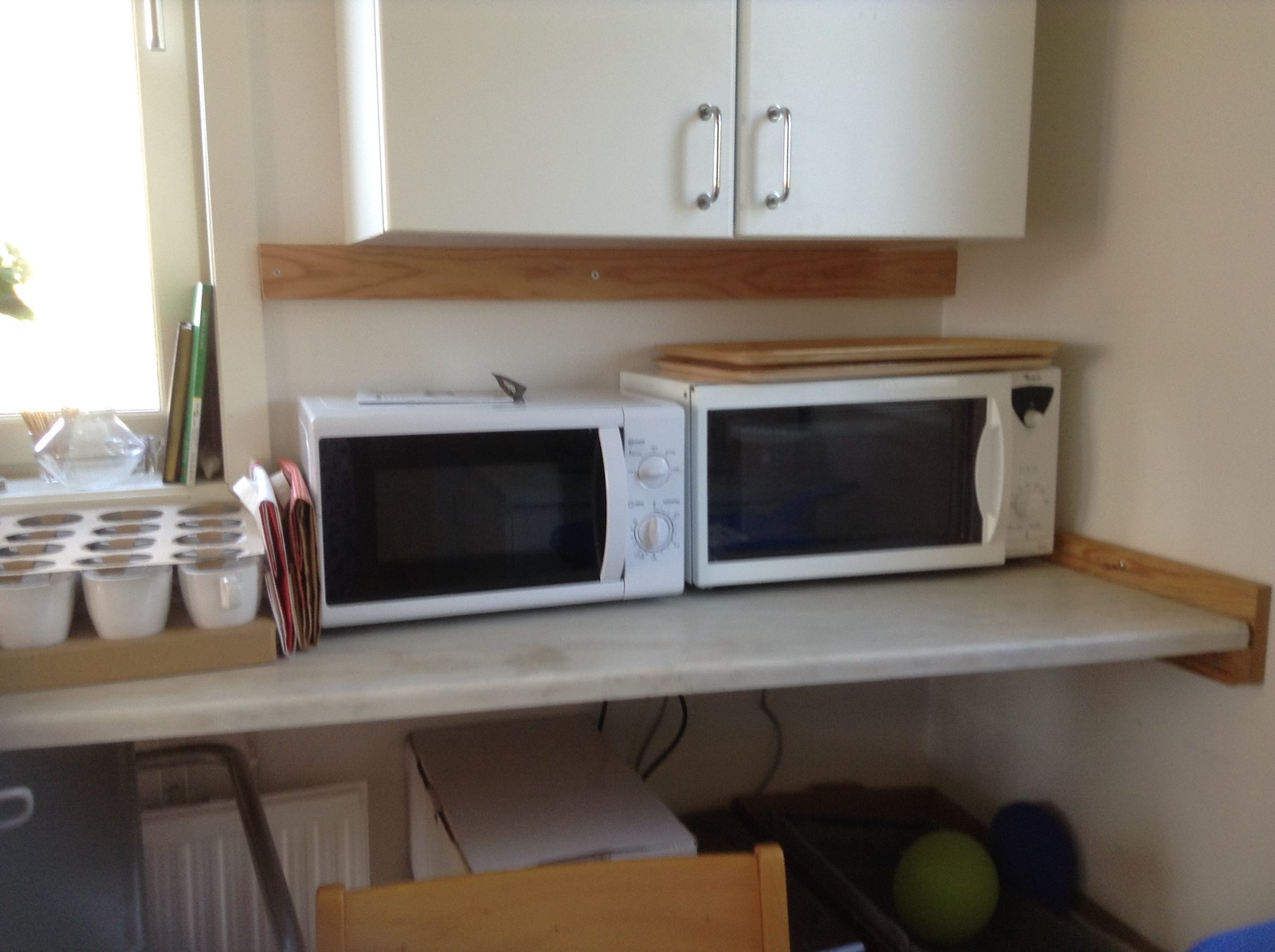This is an amateur photograph of the interior of a slightly dingy kitchen, probably taken from the kitchen table. The focal point is a white countertop, possibly marble or plastic, with two white microwave ovens. The microwave on the right is slightly larger, both have black doors with white handles, but they are from different brands. On top of the larger microwave, there are tan-colored wooden planks or serving platters. Between the microwaves, there are red and white papers and some folders. To the left of the microwaves, there is a set of at least 12 white coffee mugs neatly placed in a beige holder with a clear cover, and possibly a muffin tin on top. Above the countertop are white cabinets with silver handles and a horizontal light wood trim beneath them, running across the wall. There is a windowsill to the left, partially visible with books and some sunlight streaming through. Under the countertop, there are some unidentifiable items, including possibly a bin containing either watermelons or green cabbages, and part of a light wooden chair is visible at the bottom edge of the image. The walls are off-white, contributing to the overall white and light wood color scheme.